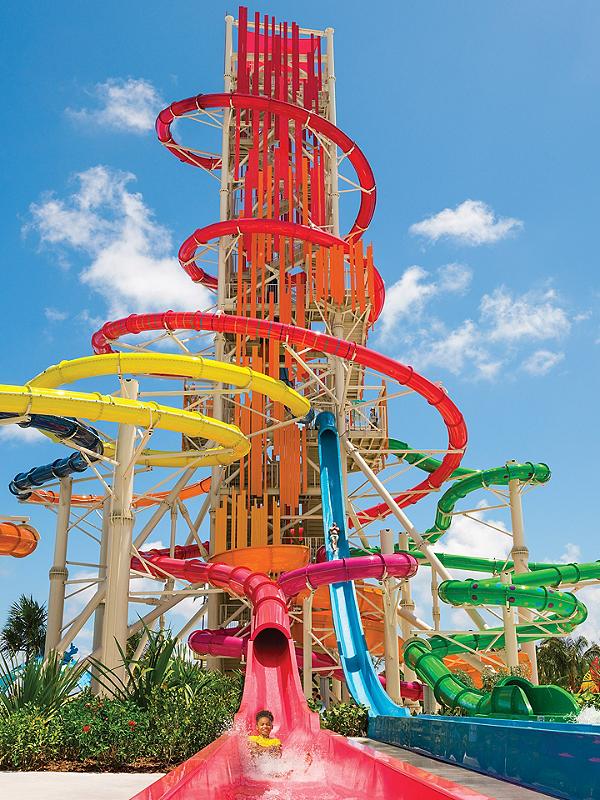The image showcases a vibrant outdoor water park, dominated by a large central tower wrapped with colorful water slides. The tower features various tubes in shades of red, yellow, green, and blue, each spiraling around before reaching the bottom. At the forefront, a black child clad in a yellow shirt emerges joyfully from the opening of a red slide, surrounded by splashes of white water. Next to them, a man descends a long blue slide, arms crossed against his chest. The scene is set against a clear blue sky dotted with white clouds, indicating a sunny day. The water park's diverse slides and the surrounding greenery, including large leafed plants and flowering bushes, add to the lively atmosphere.